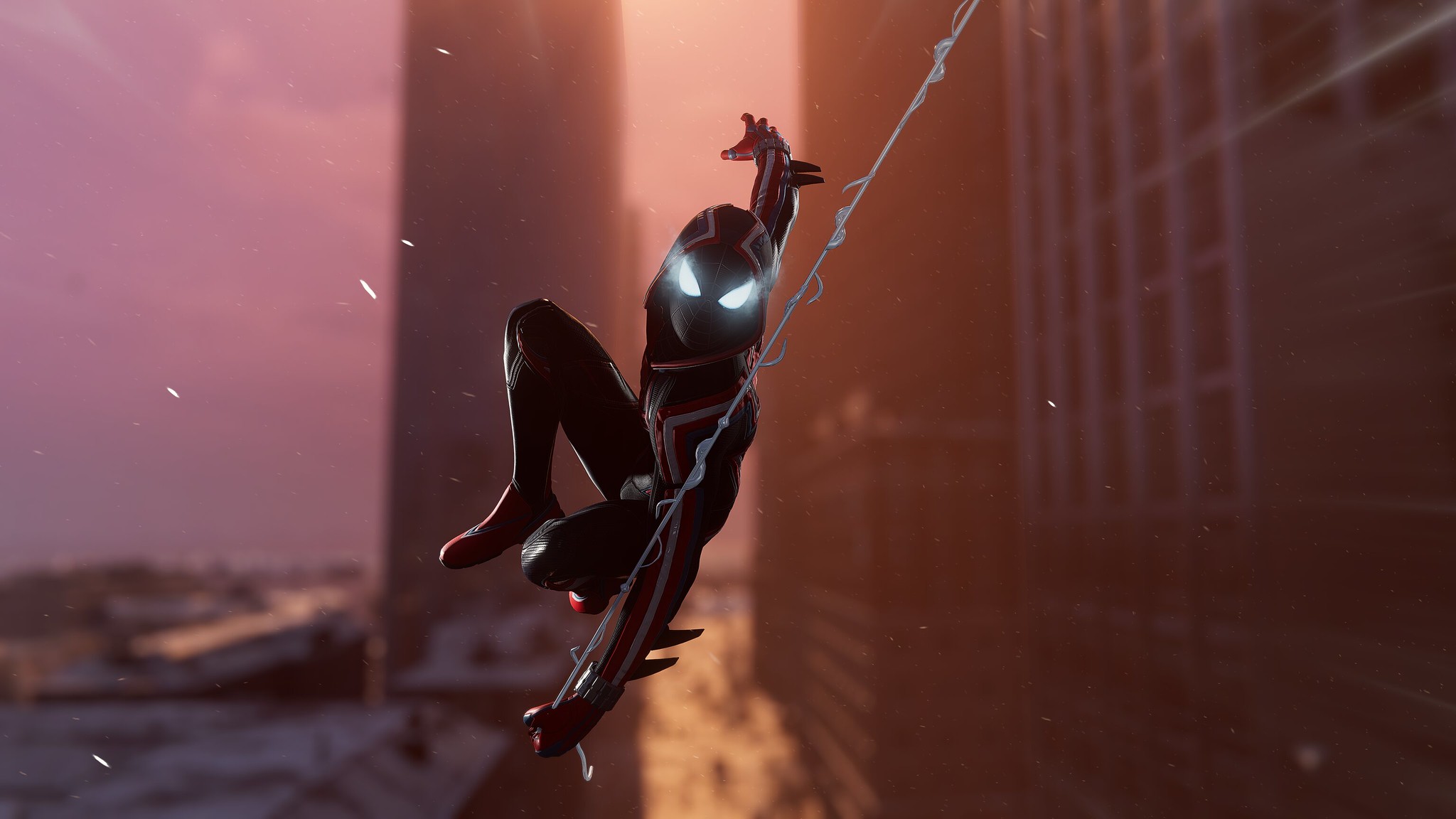This is a vibrant color image from the Spider-Man: Into the Spider-Verse animated movie, featuring Miles Morales in action. Miles is swinging through the sky on his web amidst a backdrop of numerous tall, blurred buildings against a peachy, pink, and purple glowy sunset sky. He is dressed in his distinct black Spider-Man suit with red and white accents and a hood around his mask. The head of his mask is completely black with thin, white webbing patterns, and his eyes are glowing white. His right arm is stretched out behind him, his left hand clutches the web, and his body is curled up with the right knee drawn up and left leg extended back, capturing the dynamic and agile essence of Spider-Man. The image conveys motion and energy, encapsulating a moment of gravity-defying heroism.